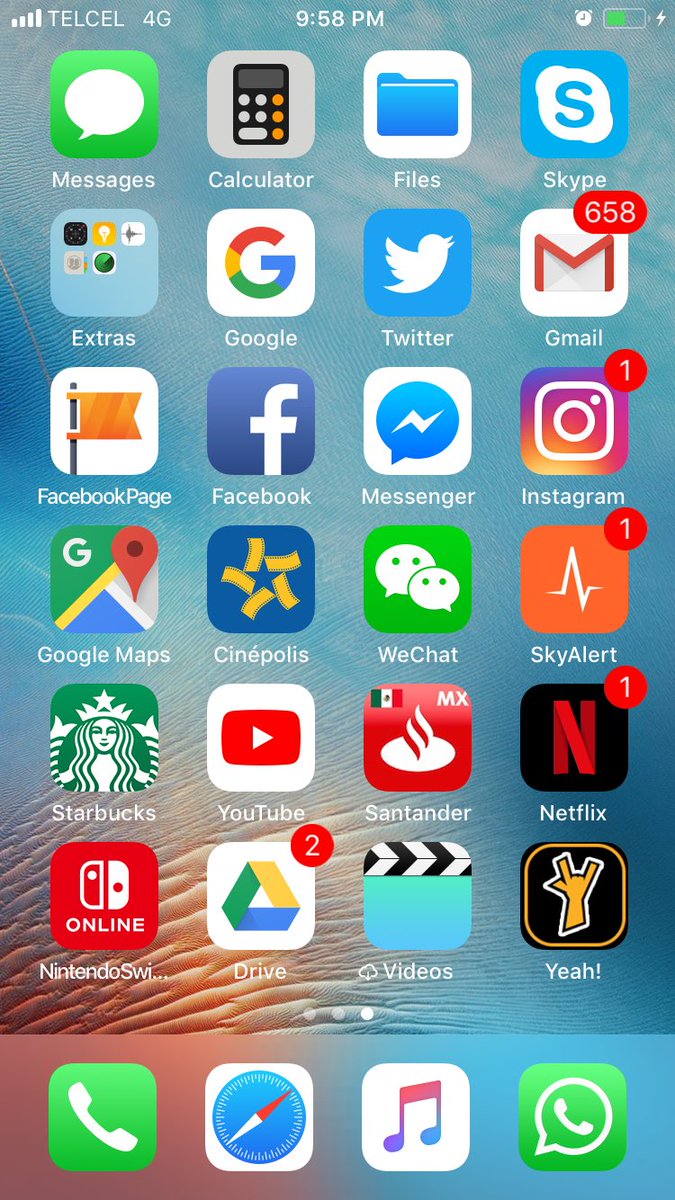This image features an Android smartphone. The background displays a gradient texture reminiscent of water or desert, transitioning from tan to a very light blue. At the very top of the screen, the status bar indicates full network signal with 'Telcel 4G'. The time is 9:58 p.m., accompanied by a clock icon and a battery icon showing the battery at 50% capacity.

The home screen shows a well-organized grid of app icons. From the top row, the apps are: 
1. Messages
2. Calculator
3. Files
4. Skype

The second row includes:
1. Extras
2. Google
3. Twitter
4. Gmail (with a red notification bubble displaying 658 unread messages)

The third row features:
1. Facebook Page
2. Facebook
3. Messenger
4. Instagram (with a red notification bubble displaying 1 notification)

The fourth row contains:
1. Google Maps
2. Cinépolis
3. WeChat
4. SkyAlert (with a red notification bubble displaying 1 notification)

The fifth row includes:
1. Starbucks
2. YouTube
3. Santander
4. Netflix (with a red notification bubble displaying 1 notification)

The sixth and final row before the dock includes:
1. Nintendo Switch
2. Drive (with a red notification bubble displaying 2 notifications)
3. Videos
4. Yeah!

The bottom dock houses four essential icons:
1. Phone
2. Compass
3. Music
4. Messenger

The notification bubbles in the top right-hand corners of certain icons indicate unread messages or notifications in Gmail, Instagram, SkyAlert, Netflix, and Drive.